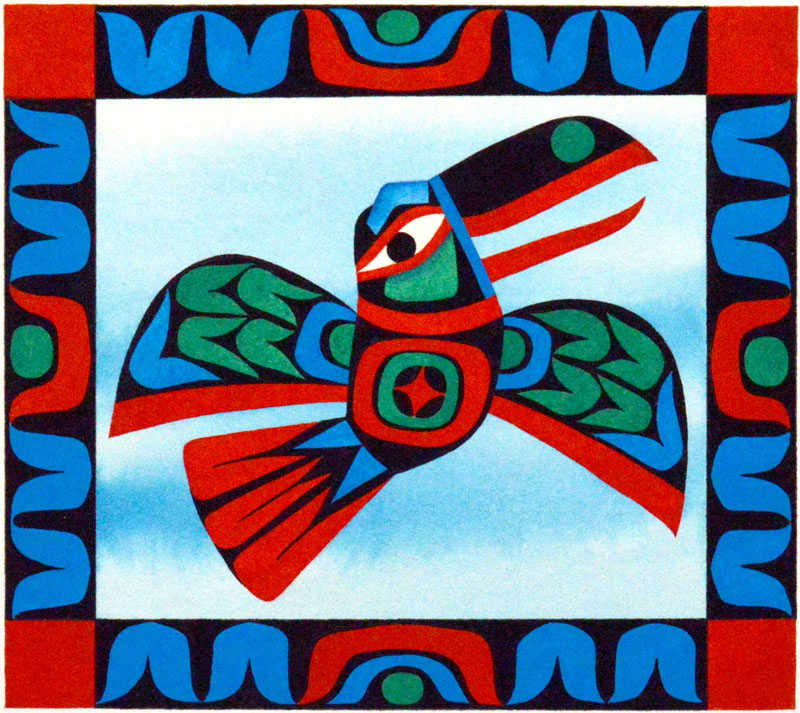The artwork is a vibrant, square-shaped, abstract illustration of a toucan mid-flight, created using various geometric shapes and bright colors, set against a blue sky background. The toucan is depicted in profile with a large, black upper beak featuring a green circle nostril and a red lower beak. Its eye is a striking white and black, rimmed with red and topped with a blue eyebrow. The bird's body is predominantly black, accented with an array of colorful geometric patterns. Its wings, spread out to the sides, are adorned with blue and green curved lines and trimmed with red edges. The tail feathers, directed towards the bottom left, showcase a blend of blue, black, and red hues. The toucan's chest features square designs in green and red. Surrounding the toucan is a tribal-like border encompassing blue, red, and black shapes, with red squares anchoring each corner, adding to the overall ethnic art style of the illustration.